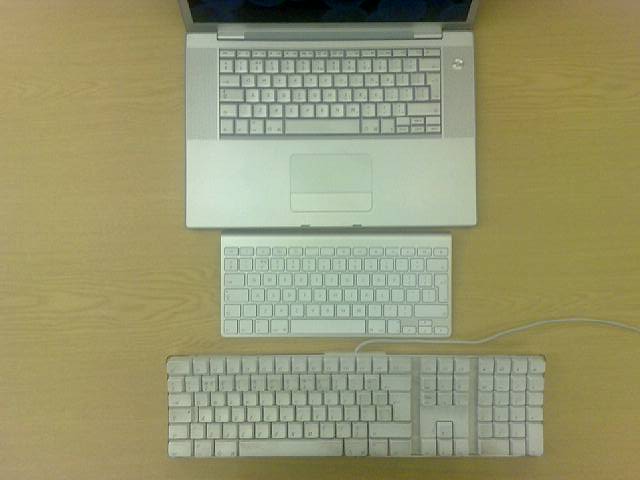The image displays an overhead view of three different keyboards arranged vertically on a light brown table. At the very top is an open laptop that resembles a MacBook Air, showcasing its built-in keyboard and trackpad. Below the laptop, there is a small, thin wireless keyboard that is likely used with an iPad or another wireless-compatible device, featuring all white keys with black letters but lacking a numeric keypad. The bottom-most keyboard is an older, wired model, possibly one of the first of its kind, with a visible cord for USB connectivity. This larger mechanical keyboard also has all white keys with black letters and includes a full numeric keypad, unlike the other two. Each keyboard reflects varying generations and types of computer input devices, providing a visual comparison of their designs and functionalities.